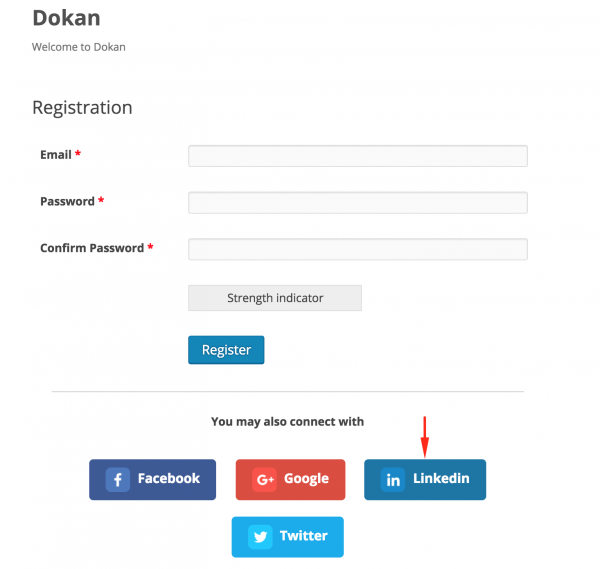In the image, there is a registration form for a website with a white background. In the top left corner, bold black text reads "TOKEA." Beneath this, smaller black text says "Welcome to Token." About an inch below, in slightly larger bold black letters, it reads "REGISTRATION." 

The form starts with a section labeled "Email" in bold black text, accompanied by a red asterisk to indicate a required field. To the right is a long, light grey rectangle for entering the email address. Beneath this, the section for "Password" follows, again in bold black text with a red asterisk. A similar light grey rectangle lies to the right for password entry. Further down, there is a section labeled "Confirm Password," also in bold black text accompanied by a red asterisk, with a corresponding light grey rectangle for input.

Below the confirm password section, there is a grey tab with the text "Strength Indicator" written in black. Further down, a blue tab reads "REGISTER" in white letters. Below this tab, a thin grey line spans across the form, separating the registration fields from the social media login options.

Underneath the grey line, small bold black text states, "You may also connect with." Here, multiple tabs for social media login options are displayed. There is a red tab labeled "Google" alongside a red square containing the white Google Plus logo. To the left, a blue tab labeled "Facebook" appears with the white Facebook logo. On the far right, there is a blue tab labeled "LinkedIn" featuring the LinkedIn logo with a red arrow pointing downwards from above.

Beneath the red Google tab is a light blue tab labeled "Twitter" in white text, accompanied by the blue Twitter logo to the left.